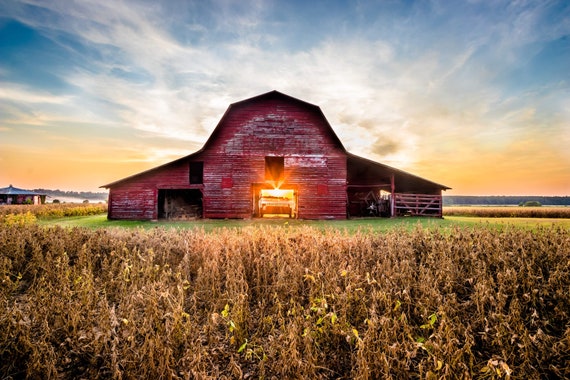In this picturesque scene set in what appears to be early spring, a weathered red barn stands prominently in a field under a vibrant sunrise. The field around the barn consists of tall, yellowish crops, possibly wheat or corn, interspersed with patches of grass and higher plants with green leaves and brown stalks. The barn itself, which is slightly run down with peeling red paint revealing white patches beneath, features a large central door through which the sun's rays are peeking, casting an ethereal glow. The sky above transitions from a warm orange and yellow near the horizon to a clear blue higher up, dotted with a few clouds. To the left of the barn, a smaller house can be seen in the background, adding to the rustic charm of the landscape. On the right side of the barn, a gated area is visible, contributing to the farm's authentic rural atmosphere.